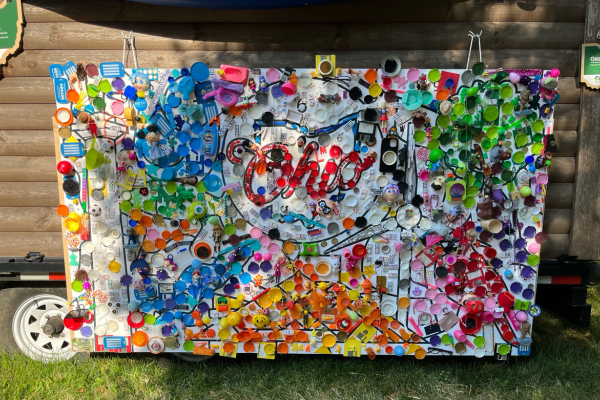The photograph captures a vibrant, handmade art piece hanging outside, centrally positioned against the backdrop of a log cabin wall and a trailer. The large, rectangular canvas, roughly the size of a blanket, is suspended by two white strings. It displays the word "Ohio" in bold, black-outlined letters, intricately formed by circular patterns and surrounded by a myriad of abstract designs in shades of red, blue, yellow, orange, green, and purple. The artwork contrasts vividly against the rustic horizontal logs of the cabin and the gray wood planks of the trailer, which is partially visible on the left side with its distinct white-rimmed tire near the bottom. In the foreground, a lush patch of green grass adds a natural element. The placement of the artwork ensures it stands out as the central focus of this outdoor scene, enhanced by the shadows suggesting an overhead tree or awning.